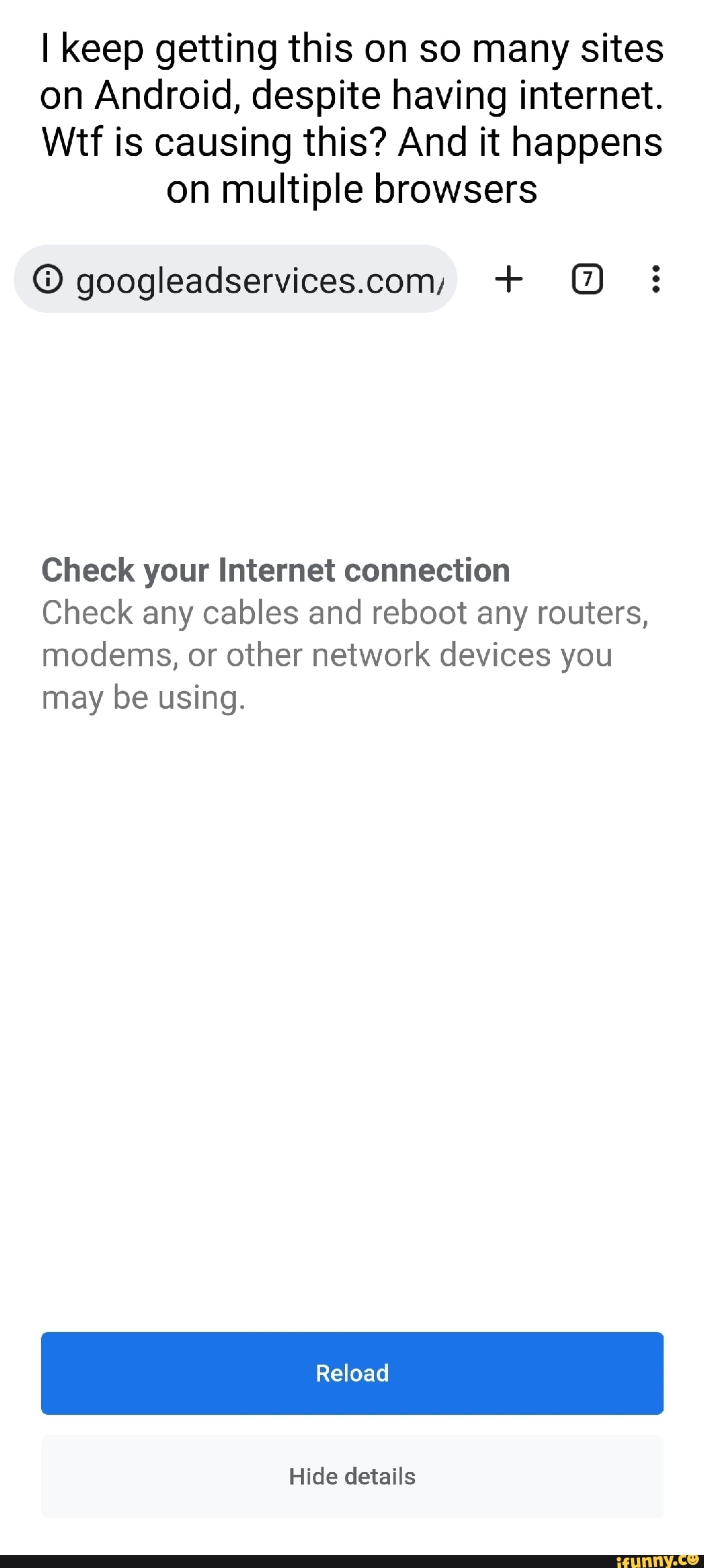The image showcases a screenshot taken on an Android cell phone, displaying an error message encountered while browsing the internet. At the top, there's a user-typed message expressing frustration: "I keep getting this on so many sites on Android, despite having internet. WTF is causing this, and it happens on multiple browsers." Below this message, the screenshot depicts a website titled "GoogleAppservices.com" with a white background and seven open tabs. 

Centered prominently is the error notification, which reads in black font: "Check your internet connection, check any cables, and reboot any routers, modems, or other network devices you may be using." At the bottom of this notification, there are two actionable options: "Reload" and "Hide the Details." The screenshot clearly illustrates the user’s issue with recurring internet connectivity errors on their Android device across multiple browsers.